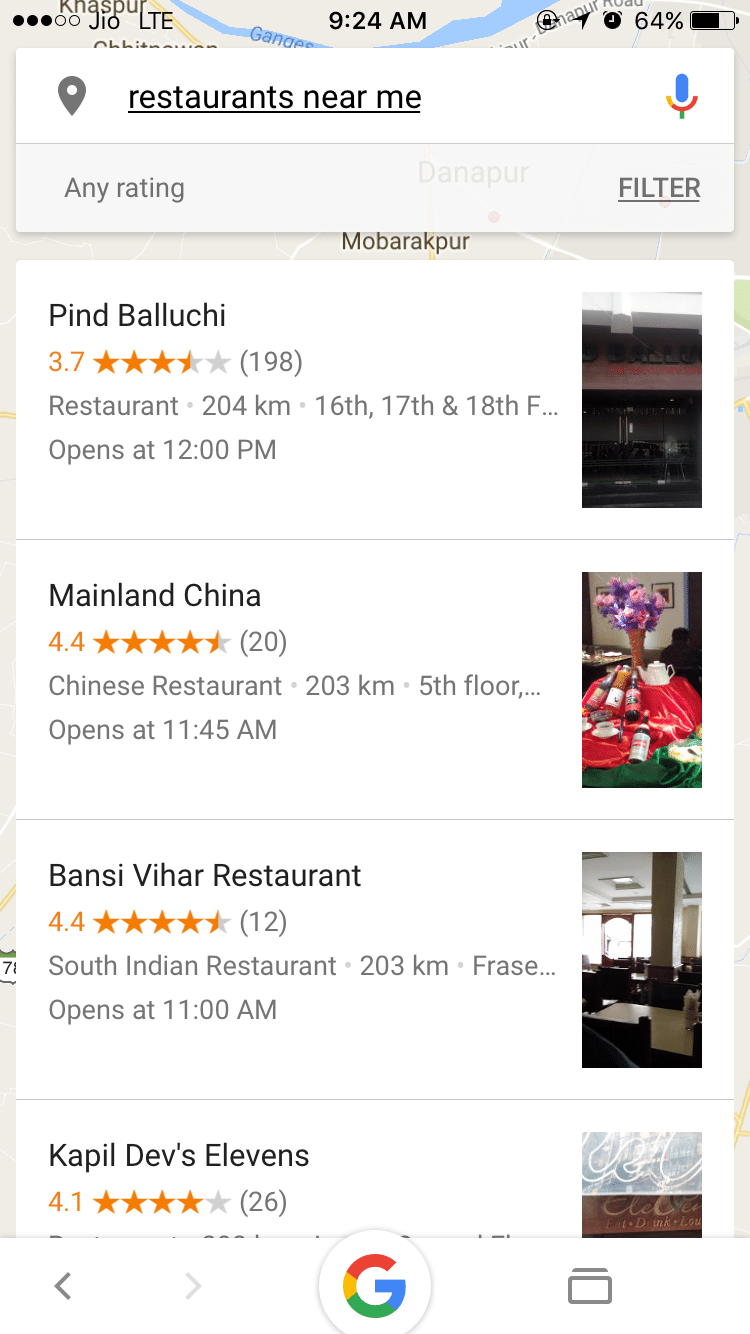A screenshot of a smartphone at 9:24 a.m. with a battery level of 64%. Below the time, there is a search box that reads "Restaurant near me," accompanied by a black location pin icon and a microphone icon. Directly beneath this, there is a filter option labeled "ANY RATING" in capital letters and underlined. The background shows a map partially obscured by a list of restaurant results. One marked location on the map is "Mobile Rockport." The listed restaurants include:

1. **Pine Belushi**: 3.7 stars from 198 ratings, located 204 km away. The address indicates it spans 16th, 17th, and 18th streets and opens at 12 p.m.
2. **Mainland China**: 4.4 stars from 20 reviews, a Chinese restaurant situated on the 5th floor, 203 km away, with an opening time of 11:45 a.m.
3. **Fancy Vihar Restaurant**: 4.4 stars from 12 reviews.